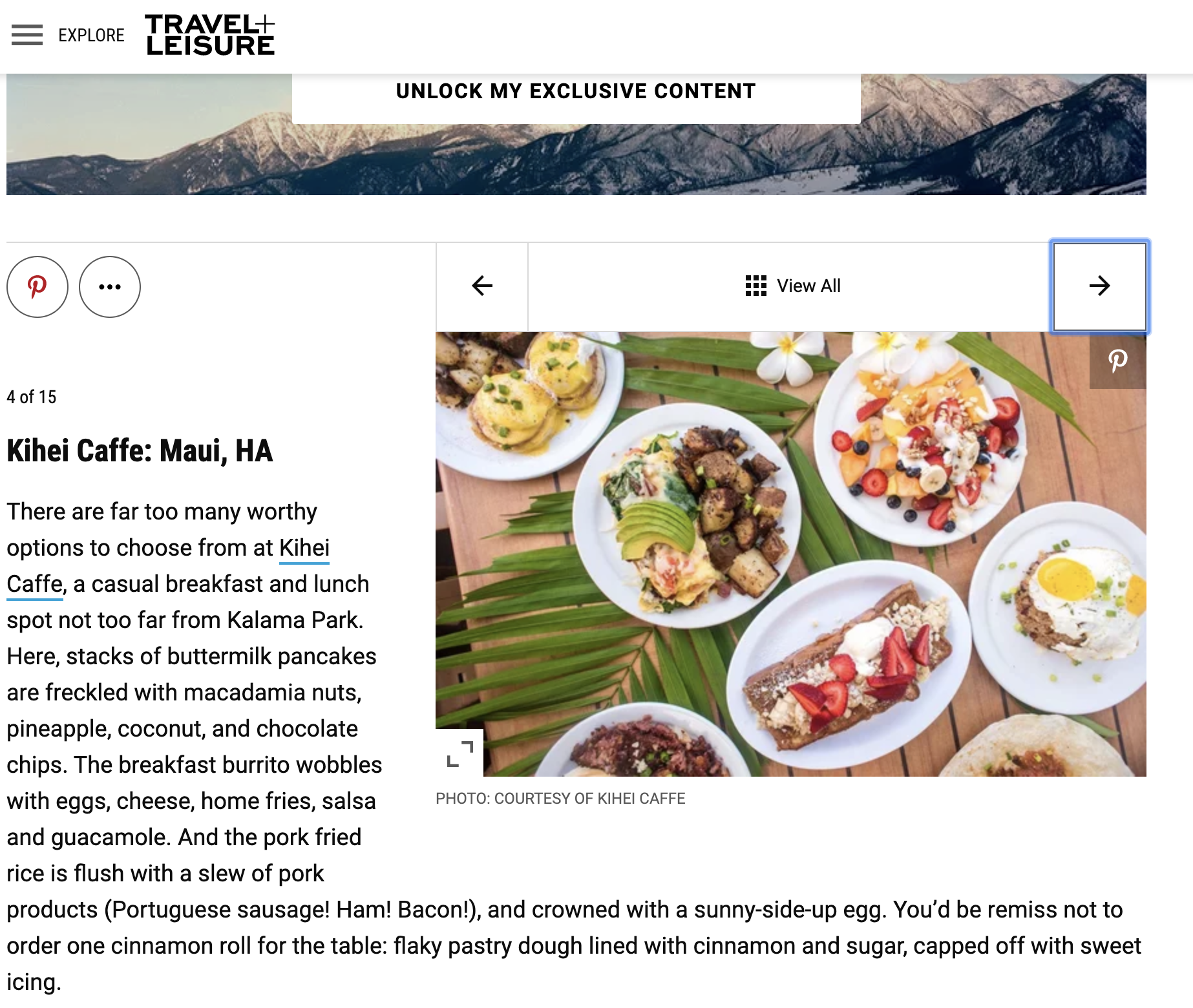On this travel webpage titled "Travel and Leisure: Explore and Unlock Exclusive Content," featuring content from Pinterest, there's a spotlight on Kehe Cafe, a cozy breakfast and lunch spot near Kalama Park in Maui. This eatery boasts an array of enticing options. Patrons can indulge in stacks of buttermilk pancakes, generously adorned with macadamia nuts, pineapple, coconut, and chocolate chips. The breakfast burrito is a hearty delight, brimming with eggs, cheese, home fries, salsa, and guacamole. Additionally, the pork fried rice is a flavor-packed dish, laden with Portuguese sausage, ham, and bacon, all crowned with a sunny side up egg. No visit would be complete without trying one of their famous cinnamon rolls.